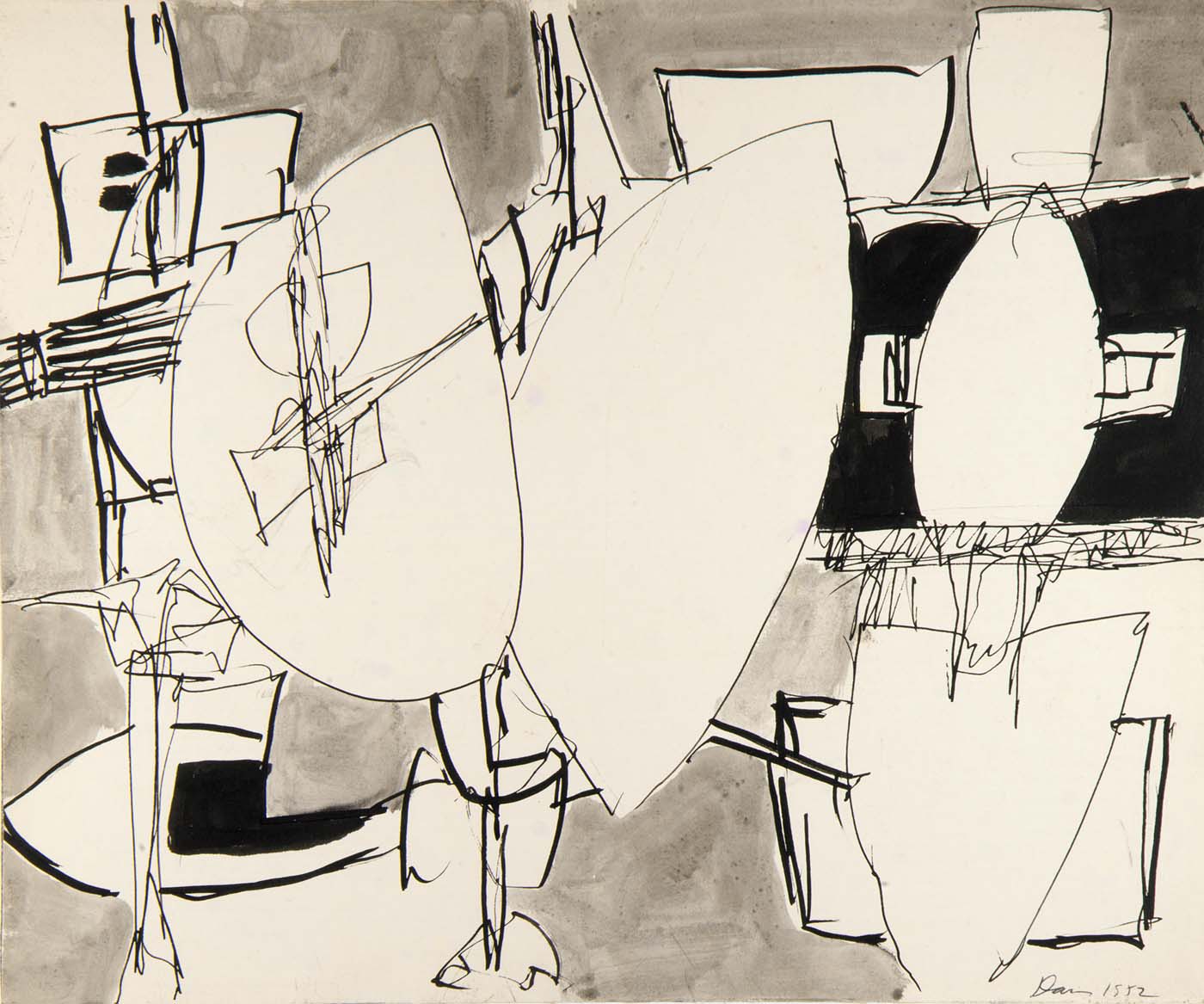The image portrays a black and white drawing that exudes an abstract aesthetic. The background is composed of varying shades of gray, appearing smudged and unevenly distributed, creating a textured canvas. The foreground displays an array of ambiguous shapes and lines sprawled across the image. These shapes defy easy categorization, though hints of crude triangles and jagged, interconnected forms suggest an attempt to depict everyday objects such as chairs or furniture, albeit in an extremely abstract manner. The drawing incorporates both thick and thin lines, contributing to its chaotic and disordered vibe, as if representing scattered thoughts. Notably, in the bottom right corner, there is a small, inscrutable signature by the artist, possibly starting with a 'D', followed by what seems to be the year '1552'. Overall, the piece gives off an impression of a quickly sketched, somewhat pretentious art piece, with elements of scattered scribbles and minimalistic gray paint, evoking a crude yet complex rendering on simple paper.